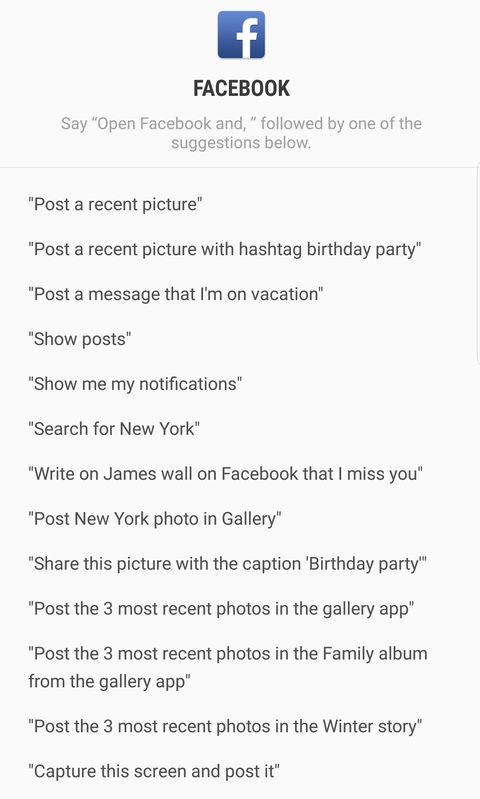This image depicts the Facebook interface. At the top, there is the iconic Facebook logo, which features a blue and white color scheme with a bold letter "F" alongside the word "Facebook" in black. Below the logo, grey text prompts the user to "Open Facebook," followed by a list of suggestions. 

The suggestions are presented in a list format with a grey background and black text:
1. Post a recent picture.
2. Post a recent picture with the hashtag #birthdayparty.
3. Post a message that says "I'm on vacation."
4. Show posts.
5. Show me my notifications.
6. Search for New York.
7. Write on James Wall's Facebook that "I miss you."
8. Post a New York photo from the gallery.
9. Share this picture with the caption "birthday party."
10. Post the three most recent photos in the gallery app.
11. Post the three most recent photos in the family album from the gallery app.
12. Post the three most recent photos in the winter story.
13. Capture this screen and post it.

The detailed descriptions provided in each suggestion give clear instructions for various Facebook functionalities, all set against a simple grey background with contrasting black text for readability.